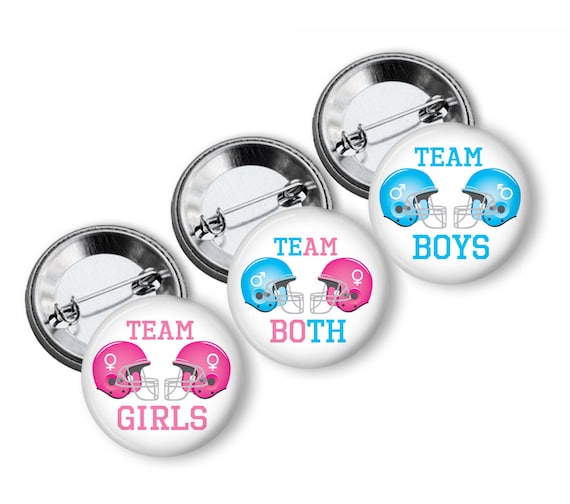The image displays a series of six badges arranged diagonally from the bottom left to the top right. There are two layers of badges: the top layer consists of three badges facing forward, while the bottom layer has three badges placed upside down, showing their stainless steel backs with pins.

On the top left badge, labeled "Team Girls," there are two pink helmets with white female symbols, one helmet on the left and one on the right. The text "Team Girls" is written in pink, with "Team" at the top and "Girls" at the bottom, all against a white background.

In the center badge, labeled "Team Both," the text is multi-colored: "TE" and "TH" are blue, while "AM" and "BO" are pink. The badge features two helmets facing each other in the middle — a blue helmet with a white male symbol on the left, and a pink helmet with a white female symbol on the right.

The top right badge, labeled "Team Boys," features two blue helmets with white male symbols. "Team Boys" is written entirely in blue, with "Team" at the top and "Boys" at the bottom.

Additionally, the reverse sides of these badges are partially visible beneath the top layer, revealing the stainless steel backs and pins of the bottom badges, which mirror the arrangement of the top layer.